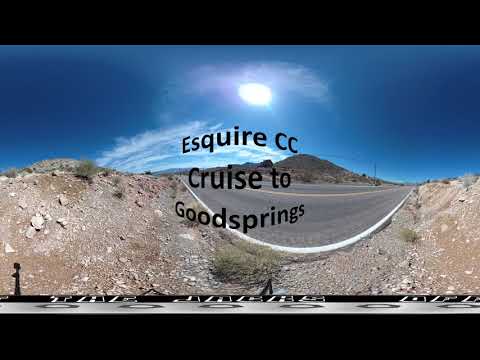The photograph captures a wide-angle, fishbowl-type view of a desert landscape. Taken from near ground level, it features a two-lane blacktop highway that curves towards the viewer, bordered by a white stripe on the edge and a yellow solid line in the center. Surrounding the road is a rocky, dirt surface with sparse, scrubby vegetation, characteristic of a desert environment. The sky above is a brilliant blue, gradually deepening in shade toward the edges, with a few wispy clouds and a bright, beating sun. In the center of the image, black text is superimposed in three rows, reading: "Esquire CC" on the first line, "Cruise to" on the second, and "Goodsprings" on the third. Below this text is a black border featuring additional text that resembles a ticker tape, though not fully legible. The scenery suggests a peaceful, laid-back moment, likely captured during a motorcycle ride across the country, offering a vivid snapshot of the arid, open landscape.